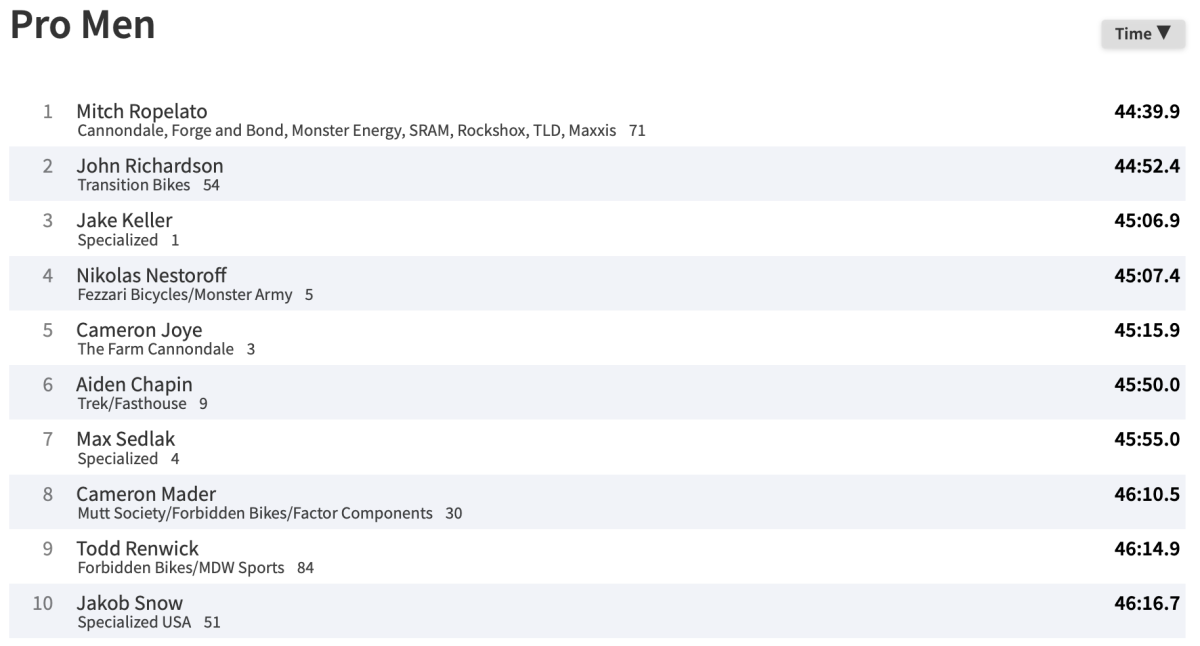This screenshot presents the leaderboard for the Pro Men category, prominently indicating the competitive times of the top ten participants. In the upper right corner, there’s a "Time" label accompanied by a dropdown menu. The competitors are listed in descending order from 1st to 10th place, with detailed affiliations and timing information:

1. **Mitch Ropelato** (Cannondale, Forge and Bond, Monster Energy, SRAM, RockShox, TLD, Maxxis 71) - *44:39.9*
2. **John Richardson** (Transition Bikes, 54) - *44:52.4*
3. **Jake Kellers** (Specialized, 1) - *45:06.9*
4. **Nicholas Nesterov** (Fezzari Bicycles, Monster Army, 5) - *45:07.4*
5. **Cameron Joy** (The Farm, Cannondale, 3) - *45:15.9*
6. **Aiden Chappin** (Trek, Fasthouse, 9) - *45:50.0*
7. **Max Sedlak** (Specialized, 4) - *45:55.0*
8. **Cameron Mater** (Mutt Society, Forbidden Bikes, Factor Components, 30) - *46:10.5*
9. **Todd Renwick** (Forbidden Bikes, MDW Sports, 84) - *46:14.9*
10. **Jacob Snow** (Specialized USA, 51) - *46:16.7*